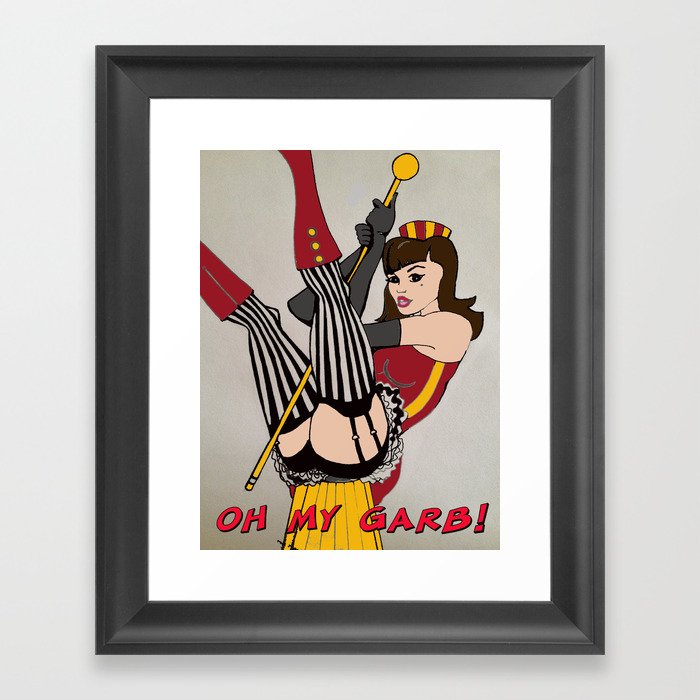This framed photograph features an artistic, cartoon-like depiction of a circus-themed woman in a playful and provocative pose. Encased in a dark gray frame with a white mat border, the image captures a fair-skinned, brunette Caucasian woman, likely in her mid-20s, with long brown hair and a beauty mark below her right eye. She wears a red and yellow striped cap atop her curls and has red lipstick enhancing her seductive expression.

The woman is dressed in a vibrant ensemble: a red and yellow corset-style top paired with black panties and adorned with red boots, each featuring three yellow buttons. Her legs are wrapped in black and white striped stockings, held up by garter belts. She also has long gray gloves extending to her upper arms. Sitting on a small yellow bucket or circular object, she holds a yellow pool cue or gold staff between her legs, with her feet kicked up in the air, adding to the whimsical and cheeky atmosphere.

The photograph includes the bold, red text "OH MY GARB!" in all capital letters under the image, complementing the playful and eye-catching aesthetic of the artwork.